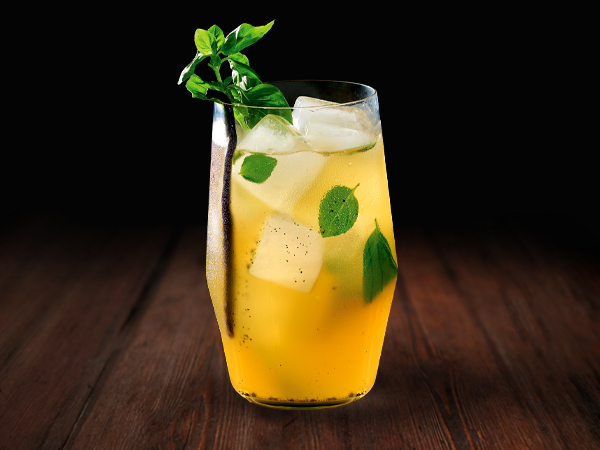This photograph captures a yellow-hued cocktail, reminiscent of a light tea or lemonade, presented in a see-through glass resting on a dark wooden table. The background is completely black, creating a striking contrast that highlights the drink. The cocktail features three visibly large, frosted square ice cubes, one of which is fully submerged while the others are partially visible at different levels within the glass. Scattered throughout the beverage are small black specks, potentially pepper or vanilla bean pods, which have also settled at the bottom. Floating amidst the ice cubes are multiple mint leaves, adding a fresh, green accent to the composition. Additionally, a prominent sprig of mint, with a brown stem and lush green leaves, extends from the left side of the glass, draping over the rim. The overall aesthetic is simple yet elegant, with the dark wood and black background enhancing the vibrant details of the cocktail.